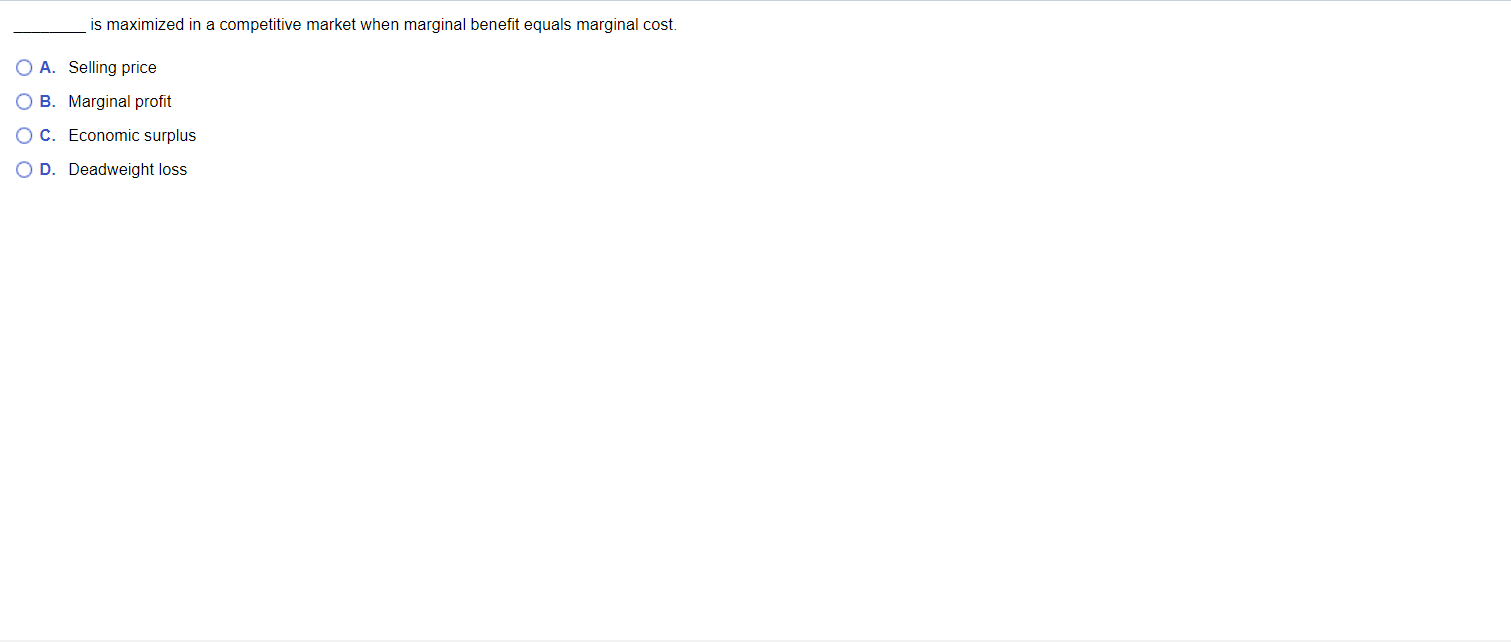This is a screen capture of a multiple-choice question displayed on a white background. The text is presented in black font with four answer options labeled A, B, C, and D. Each label (A, B, C, D) is encased in a blue circle with a blue outline. The question reads, "____ is maximized in a competitive market when marginal benefit equals marginal cost." The four answer choices are as follows:
- A: Selling Price
- B: Marginal Profit
- C: Economic Surplus
- D: Deadweight Loss

Additionally, the screen is minimalistic, with nothing else visible except for thin, faint grey lines at both the top and bottom of the screen. The overall design is clean and straightforward, emphasizing the multiple-choice question.